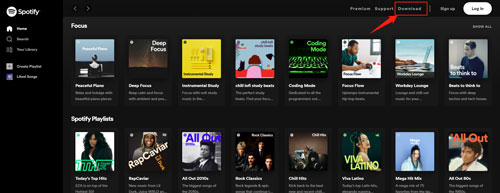The image is a horizontal screenshot from a smartphone device, likely captured from the Spotify app interface. On the left side, there's a solid black vertical panel featuring a small circular icon at the top, followed by the text "Spotify." Below this, the panel includes a "Home" button and several other icons such as "Your Library," "Create Playlist," and "Liked Songs." The overall color scheme of the panel is a combination of dark gray and black.

On the top right of the image, there are navigational arrows for going forward and backward. Adjacent to these controls, there are options for "Premium," "Support," and "Download," with the "Download" option highlighted by a red box and a red arrow pointing to it. Below these, a gray "Sign Up" button and a white "Log In" button are visible.

The central portion of the image showcases album covers arranged in two rows of eight, making a total of sixteen album covers. Each album cover is accompanied by its title in white text and additional information in gray text beneath it, though this text appears blurry.